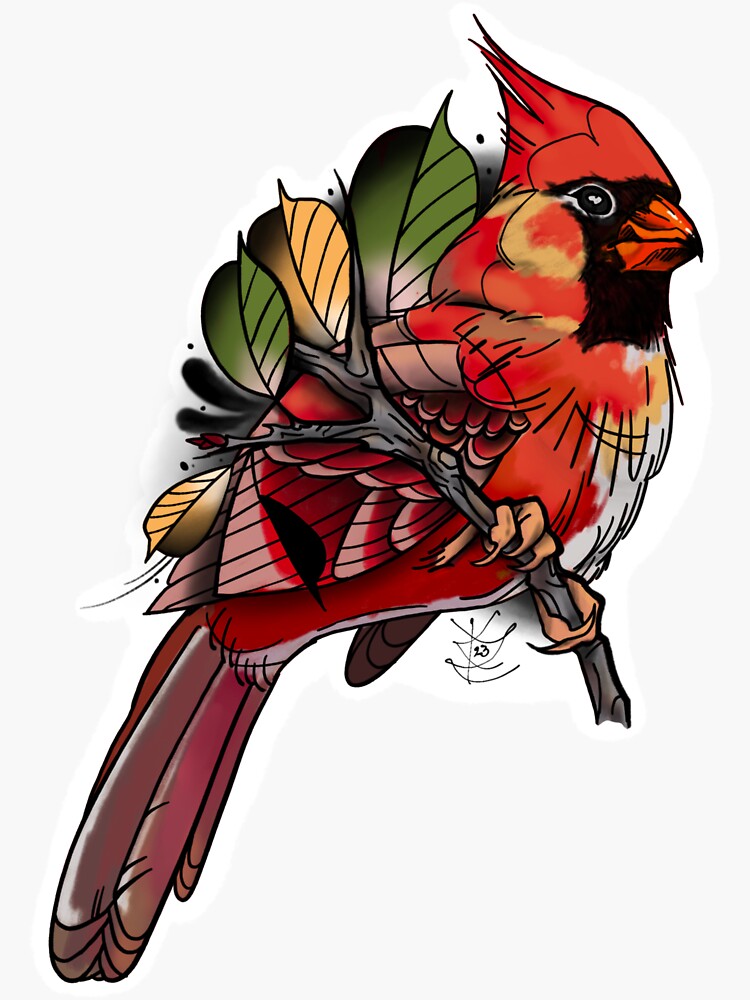The image depicts a detailed and vibrant watercolor or digital illustration of a cardinal perched on a branch, which could also be seen as stylized art similar to a tattoo stencil. The bird, showcasing a striking red and orange palette, sports a sharp crested mohawk-like head with a contrasting orange beak and a black mask around its face. The tail feathers feature a subtle purple hue and lighter shades towards the bottom. Its beige claws grip the gray branch firmly, which is accented by strong black line art and adorned with two green and two yellow leaves. The bird faces right, presenting a full profile, including its distinctive white face and yellow chest markings. The background is completely white, emphasizing the cardinal's vivid coloration. Additionally, there is an artist's signature beneath the bird, adding a personal touch to the illustration.